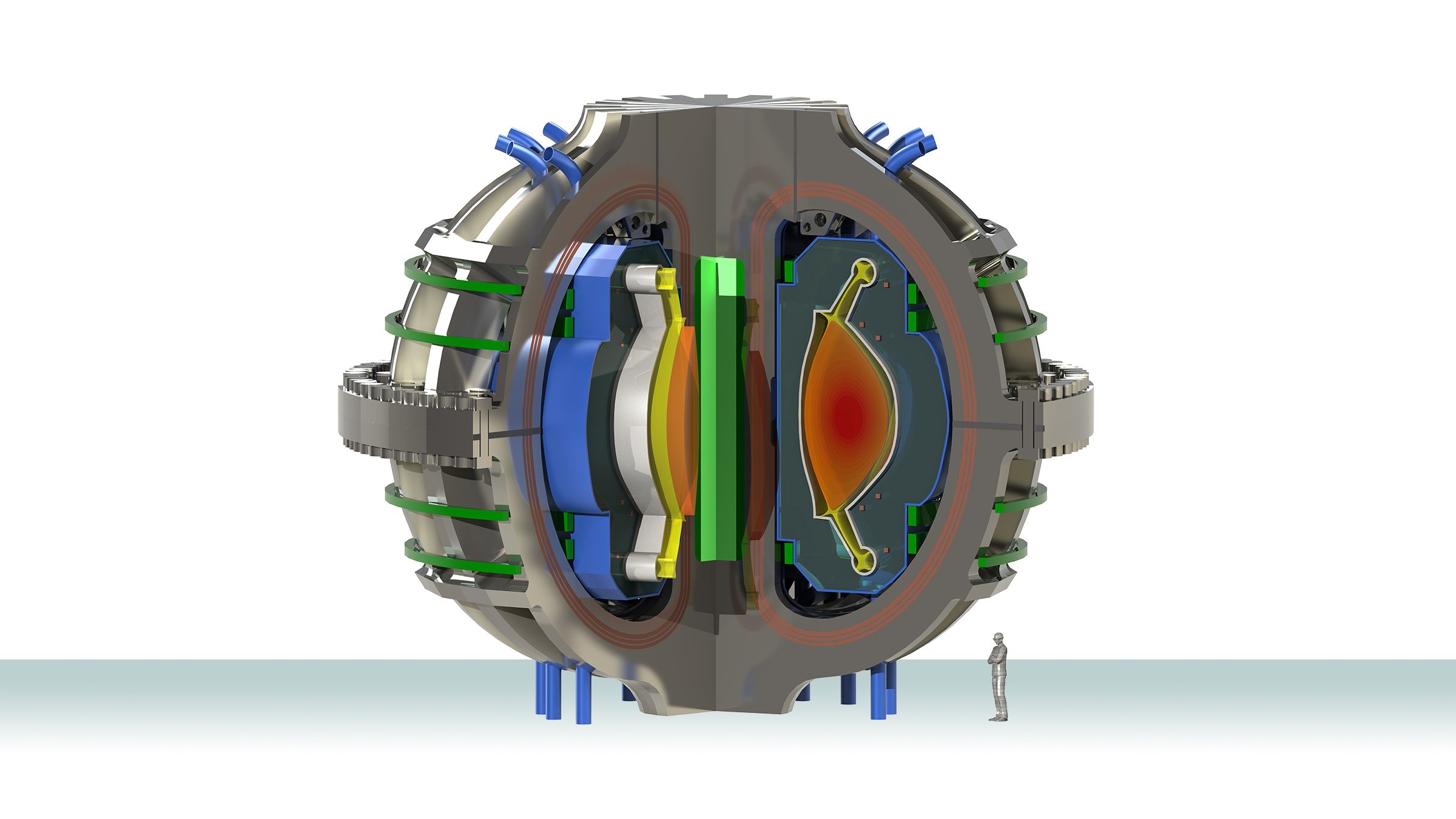This image is a detailed digital illustration of a large, spherical mechanical device, showcasing both its exterior and intricate internal components. The outer surface is a blend of gray, blue, and green metallic hues, accented by two bright Kelly green bands running parallel to the equator. A prominent thick band circles the orb’s midsection, seemingly holding it together. Attached to the device are small blue metallic legs and bright electric blue exhaust pipes protruding from the top, neatly aligning along the orb’s axis.

The illustration reveals a cross-sectional view of the device, sliced in half to expose its internal mechanisms. The inside components are vividly colored in a palette of red, orange, white, yellow, and various shades of blue. These segments are intricately arranged in layers, resembling a beanie cap with extensions on either side, stacked meticulously within the spherical structure. 

In the background, the image is set against a predominantly white space with a light blue and green-toned foreground, enhancing the mechanical device’s prominence. To the left, a small figure of a person stands in a silver spacesuit with their arms crossed, highlighting the immense scale of the orb. The entire scene is framed within a rectangular format, providing a comprehensive view of this elaborate mechanical or possibly nuclear contraption.